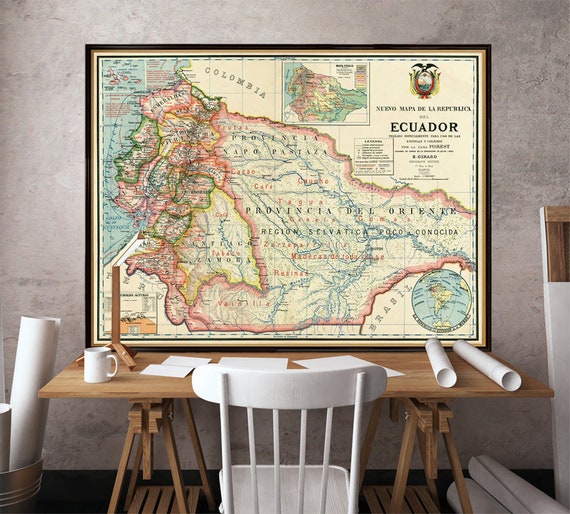In the center of the room, atop a plain brown wooden desk, lies an aged, olive-colored map titled "Nuevo Mapa de la Republic Ecuador." This detailed map of Ecuador showcases its borders, with Colombia to the north, Brazil to the southeast, Peru to the west, and the Pacific Ocean lining its coastline. The map appears to be framed in black wood and features various colors indicating the country's topography. Surrounding the desk are multiple white paper rolls, some scattered on the tabletop, others tucked into a metal bucket to the left, and a few resting on the floor to the right. The scene is set against a grey wall backdrop, with an empty white chair positioned in front of the desk. Additional details include a white coffee mug among the papers on the desk, suggesting a workspace dedicated to cartography and study.